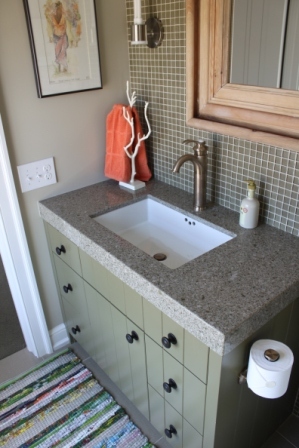A charming section of a modern bathroom featuring a sleek vanity is captured. The overall color scheme is a palette of grays. The backsplash behind the vanity showcases a mosaic of small square gray tiles with contrasting white grout, lending a sophisticated touch to the space. Mounted on the wall is an elegant lamp with a dark metal base, designed to appear as though it houses a candle, adding a warm, ambient glow.

The vanity itself is a contemporary rectangular piece, finished in a polished gray material, likely granite, which complements the deep rectangular sink it houses. The sink boasts a brushed silver high-arc faucet adding a modern flair. Sitting on the countertop is a white soap dispenser with a pump, alongside a small decorative white tree, adding a touch of nature-inspired decor.

To the left of the vanity, the wall is painted a light gray and adorned with a watercolor painting whose specifics are indistinguishable but adds an artistic element. The frame of the mirror above the vanity, appearing to be light wood, enhances the bathroom's cozy aesthetic.

The vanity is functional with ample storage: one central door with black knobs houses the main compartment, flanked by three drawers on each side. Below, a woven rug with patterns of green, pink, and gray gives a pop of color and comfort. Nearby, the toilet paper holder is uniquely upright, adding to the charm. An orange hand towel and bath towel bring a bright, warm contrast to the otherwise cool-toned room.